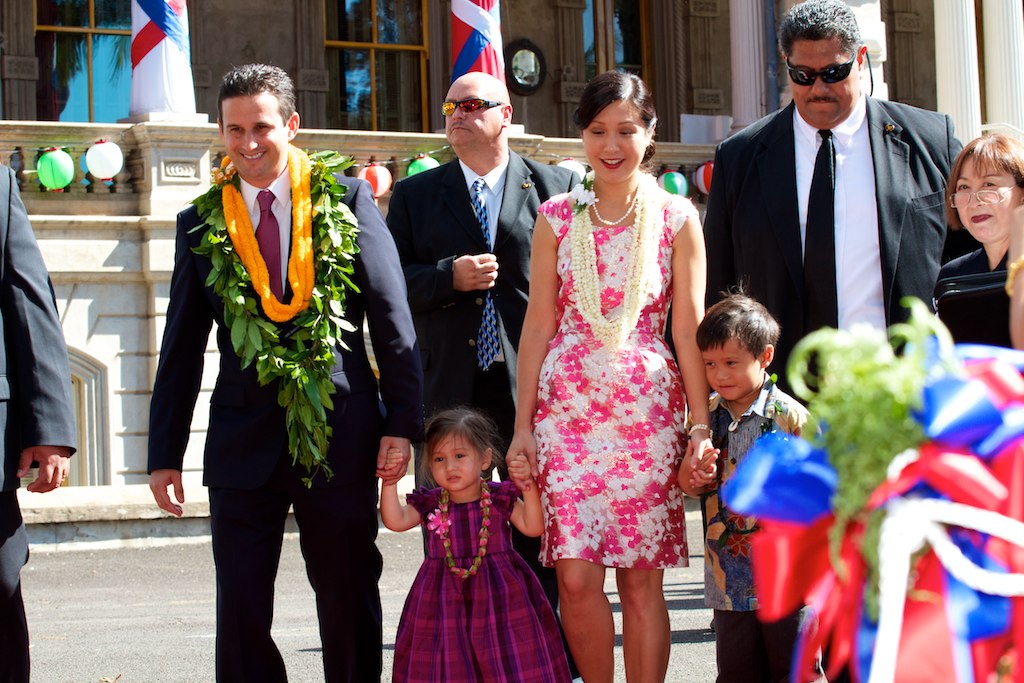In an outdoor setting, a family stands together with a few additional individuals in the background. At the center, a woman with black hair pulled back is dressed in a pink and white floral dress and wears a white Hawaiian lei around her neck. Flanking her on either side are a little boy and girl, both with dark hair and leis around their necks. The boy is dressed in a colorful shirt and black trousers, while the girl wears a purple dress with a rose garland.

To the left, a man, presumably the father, is dressed immaculately in a black suit, white shirt, and red tie. He has short brown hair and wears two yellow scarves and a green, leafy wreath. He is holding the little girl's hand, symbolizing their close connection. Positioned behind the little girl, between the man and the woman, is a bodyguard. He is a white male wearing mirrored sunglasses, a black suit, a white shirt, and a blue and black tie, adding an element of security to the scene.

To the far right of the image is another man dressed similarly in a black suit, white shirt, and black tie, also wearing black sunglasses. An Asian woman with light brown short hair, clear-framed glasses, and a black top stands nearby, adding to the group of observers. Other people can be seen in the background, adding to the lively atmosphere of the gathering in front of a building.